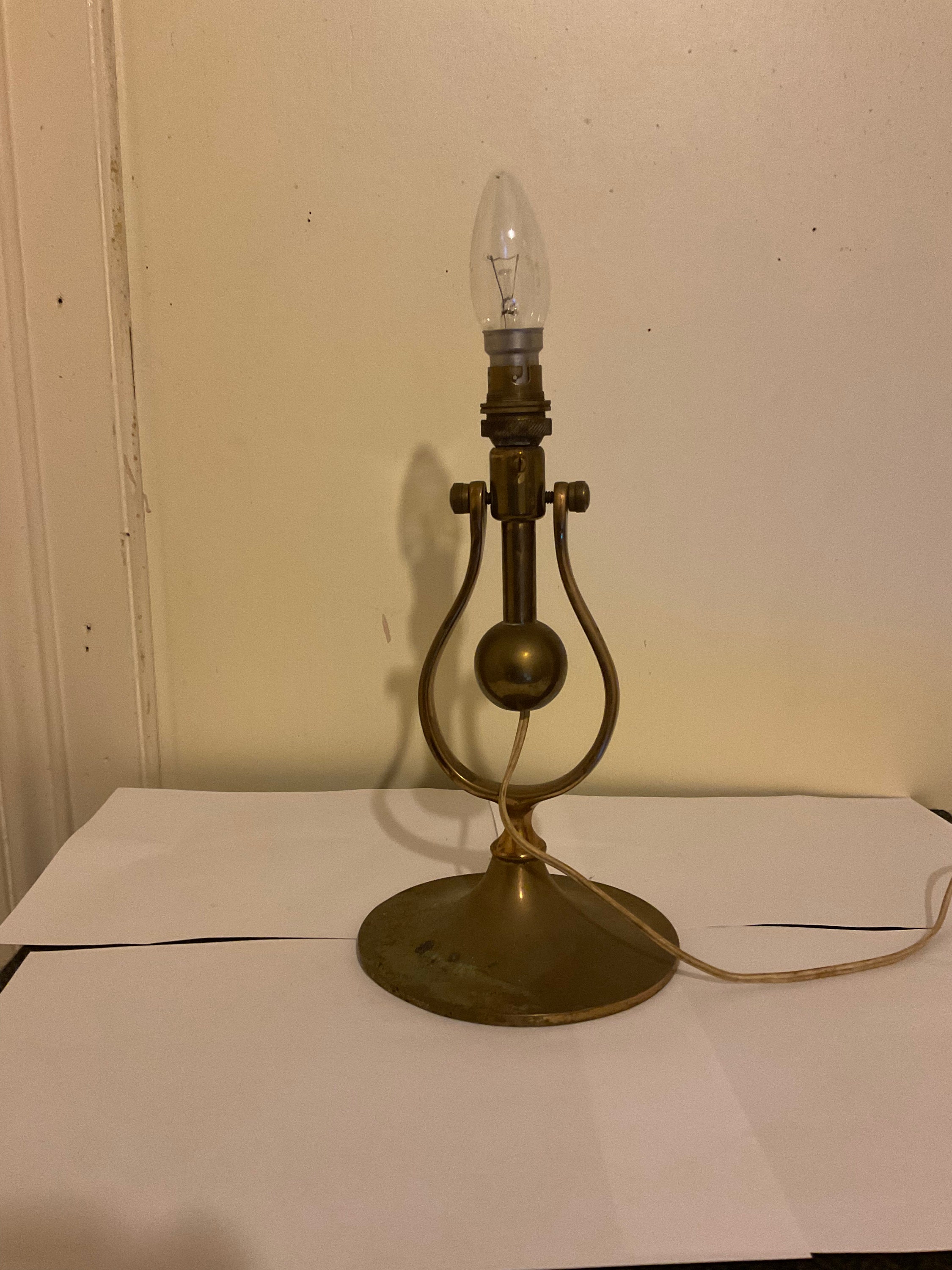The image depicts an antique brass lamp with a single small bulb resembling those found in chandeliers. The lamp base is a disc from which a cylindrical rod extends upward, branching into two arcs that hold the bulb receptacle in the middle. The lamp has no lampshade, and an aged electrical wire protrudes from the bottom. This ornate, golden metal lamp with its distinct shape and worn appearance rests on four layers of white computer paper atop a dark tabletop. The background features an old, slightly dirty white wall with visible dings and dust, alongside the trim of an entryway. The setup suggests that the photograph might be intended for insurance or selling purposes, emphasizing the lamp's antique quality by providing a clean white surface and backdrop.